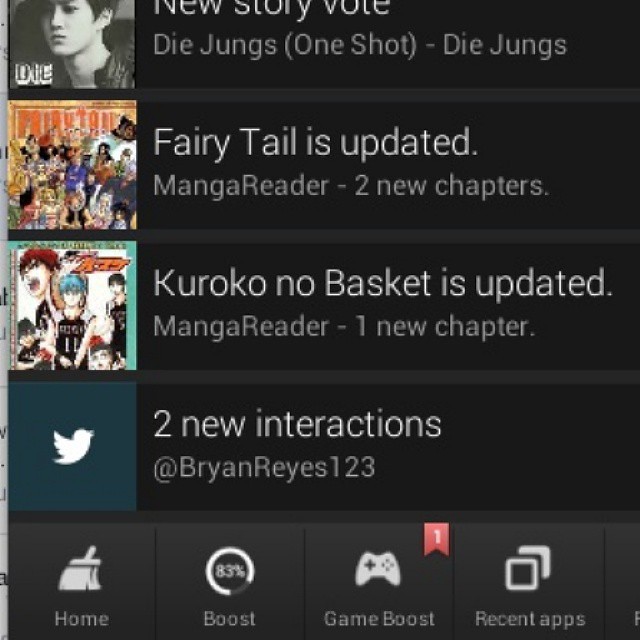The image appears to be a screenshot of a phone's home screen displaying various updates and notifications, segmented into four horizontal sections. At the top, there's a partially cut-off banner that reads "New Story Vote," accompanied by a picture of an individual facing forward on the left. To the right of the image, the text reads "Dai Jung's one-shot - Dai Jung's." Below that, a cartoon-like picture is paired with a black rectangle stating, "Fairy Tale is updated. Manga Reader, two new chapters." 

Further down, another colored, cartoonish image announces, "Kuroko No Basket is updated. Manga Reader, one new chapter." Below this, the Twitter logo can be seen, with a notification indicating, "Two new interactions at Brian Reyes 123" in a black rectangle. Finally, at the bottom of the image, there are four icons on a gray background: a house symbol labeled "Home," an icon with "Boost" indicating an 83% status, a controller labeled "Game Boost" with a '1' ribbon, and an "app widget" symbol titled "Recent Apps."

This detailed layout clearly represents the updates and interactions on the phone, showing notifications related to manga updates, social media interactions, and system functions such as boosting performance and accessing recent applications.